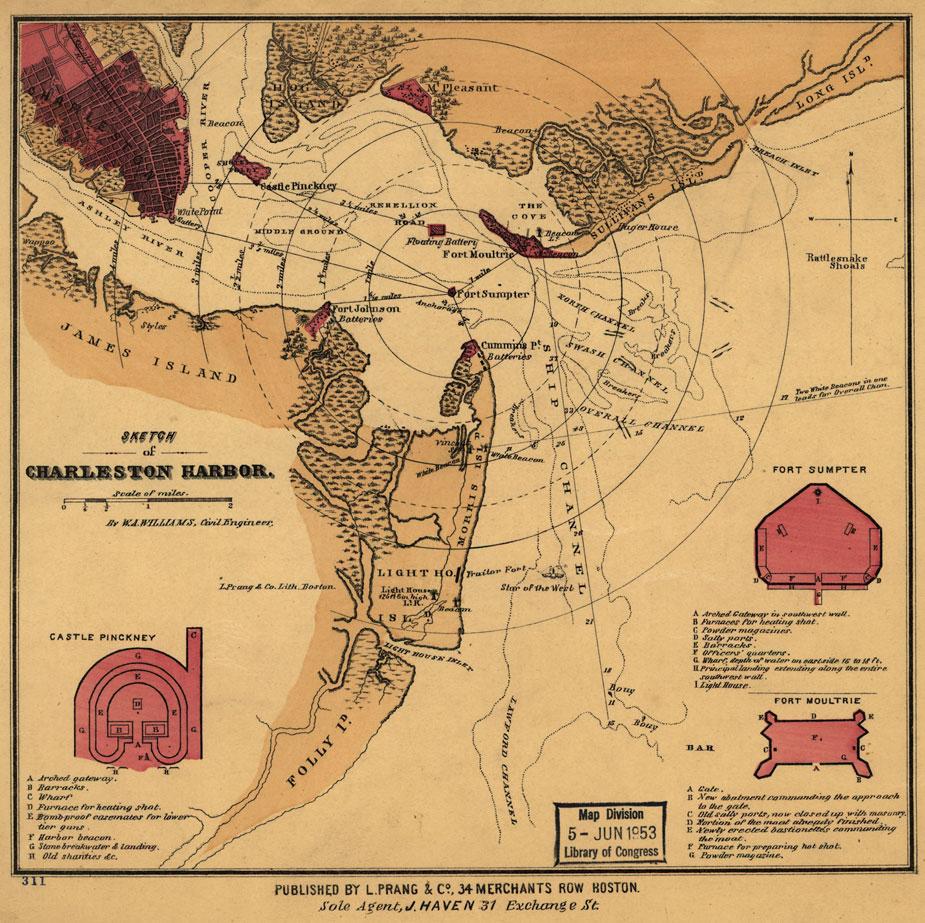This detailed illustration depicts a historical map of Charleston Harbor, primarily showcasing Fort Sumter as its focal point. The map, characterized by various shades of tan and accented with reds, highlights significant landmarks such as Fort Moultrie, Castle Pinckney, and James Island. There is a prominent stamp indicating the map was produced by the Map Division of the Library of Congress on June 5th, 1953. The left side of the image bears the title "Sketch of Charleston Harbor" along with the name of the cartographer, W. A. Williams, a civil engineer. Produced and published by L. Prang and Company at 34 Merchant Row, the image combines both illustrative and historical elements, creating an educational resource that maps out the intricate layout of Charleston Harbor and its surroundings.